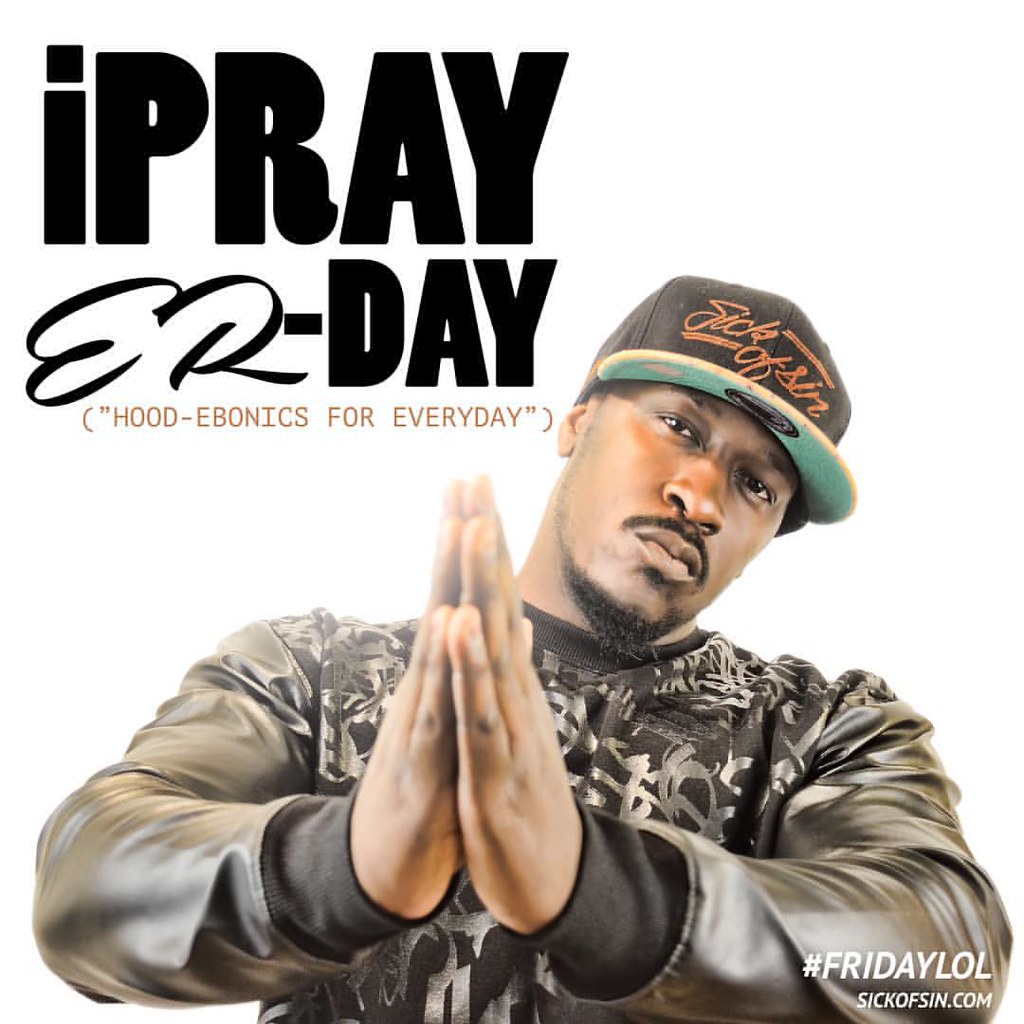The image presents what appears to be an album cover with a predominantly white background. At the center is a black man looking directly at the camera, his hands clasped in a prayer gesture in front of him. He's wearing a black baseball cap with orange lettering that reads "Sick of Sin," and the underside of the brim is turquoise. His top features black leather sleeves, while the chest area showcases a graffiti-style print.

At the top left of the image, large black letters spell out "I PRAY ER DAY," with "I" being lowercase, "PRAY" in all caps, and "ER" in a script font, while "DAY" reverts to regular all-caps. Below this phrase, in small brown letters within parentheses, it says "(Hood-Ebonics for every day)." In the bottom right corner, the text "#FridayLOL SickOfSin.com" is displayed in white.